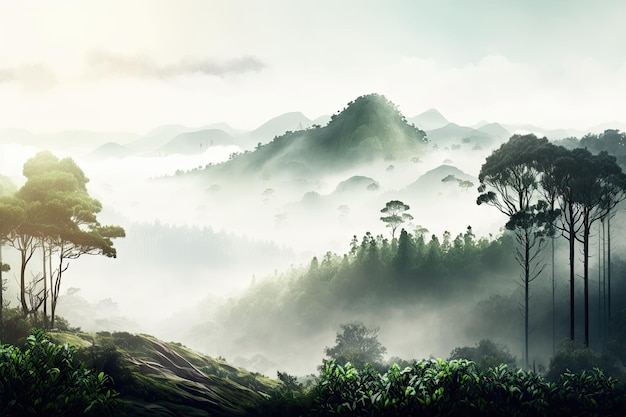This is an intricately detailed, Asian-inspired painting showcasing a serene mountain landscape enveloped in mist and fog. The scene is set from a perspective that looks across a valley towards a range of green and gray mountains, their bases obscured by the thick mist. The sky above is a blend of blue with patches of white and gray clouds, adding to the tranquil ambiance. 

In the bottom right corner stands a group of tall trees, distinguished by their slender, elongated trunks and leafy canopies that cluster at the very top. On the bottom left, a hill is adorned with shorter trees and rocky outcroppings, while mid-ground depicts a series of trees partially veiled by the mist. The foreground features some bushes and green leaves, adding layers to the composition. 

The landscape slopes downward into the valley and ascends again towards the mountains, creating a mystical atmosphere as if one is peering through the mist into a hidden, tranquil world. The overall effect is both tranquil and mystical, with no text to interrupt the natural beauty portrayed in this poetic scene.